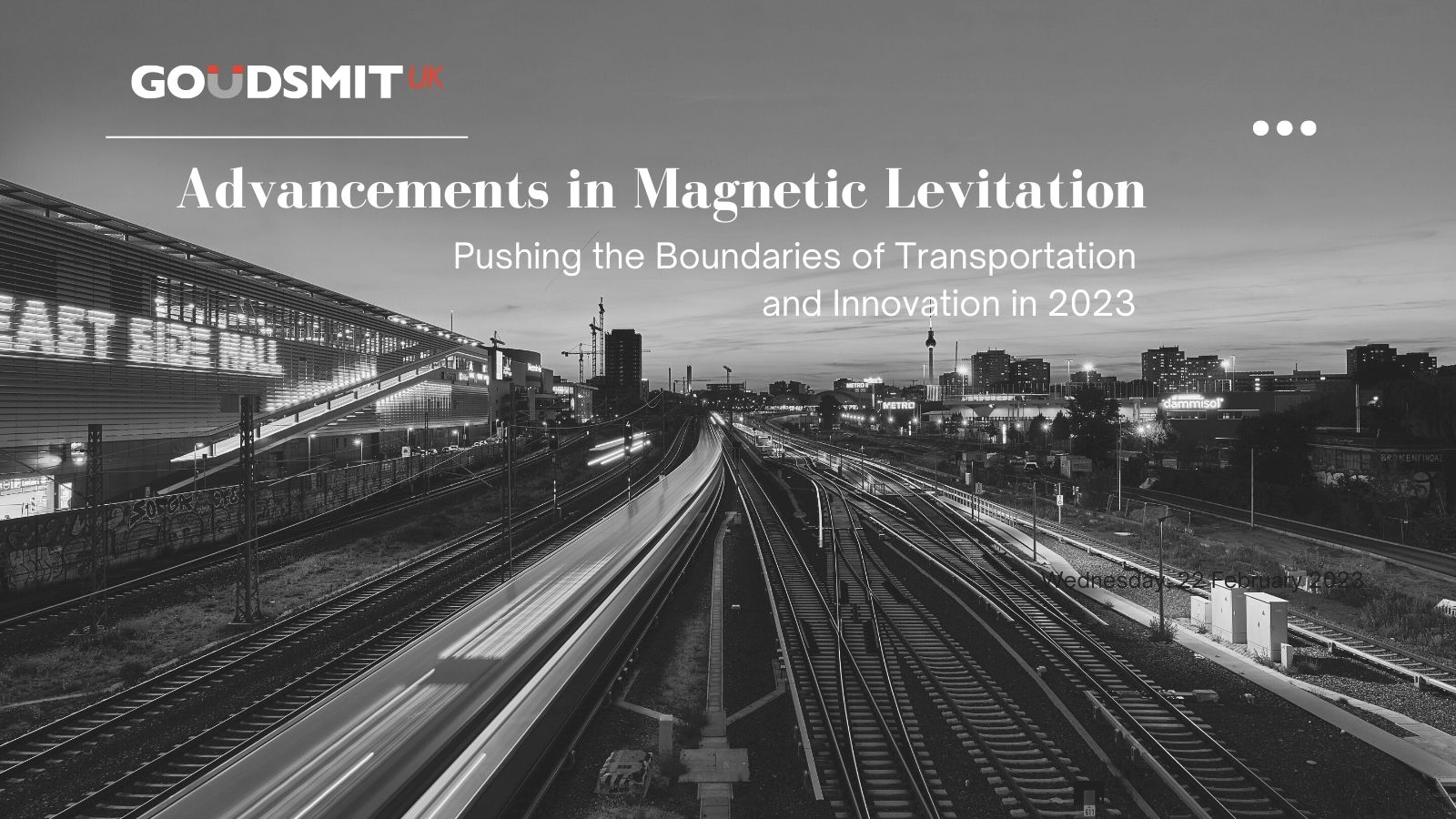The black-and-white photograph captures a sprawling rail yard set against a cityscape at dusk. Several train tracks, both modern and older, stretch out from the foreground towards a distant vanishing point. To the left, an elevated section of the tracks looks down on another track below. The city, blurred but discernible in the background, features a mix of taller and shorter buildings illuminated by faint lights. 

Prominently, on the left side of the image, stands a low, long building labeled "East Side Mall." 

The upper left corner of the photo bears the logo of Goudsmit, a company specializing in magnetic levitation technology. The name "Goudsmit" is cleverly designed with a dark gray 'U' shaped like a horseshoe magnet, featuring red tips, underlined by a thin white line. Below the logo, the text reads "Advancements in Magnetic Levitation," followed by "Pushing the Boundaries of Transportation and Innovation in 2023."

Gray skies loom overhead, casting a muted tone over the scene, emphasizing the industrial and innovative theme of the photograph.